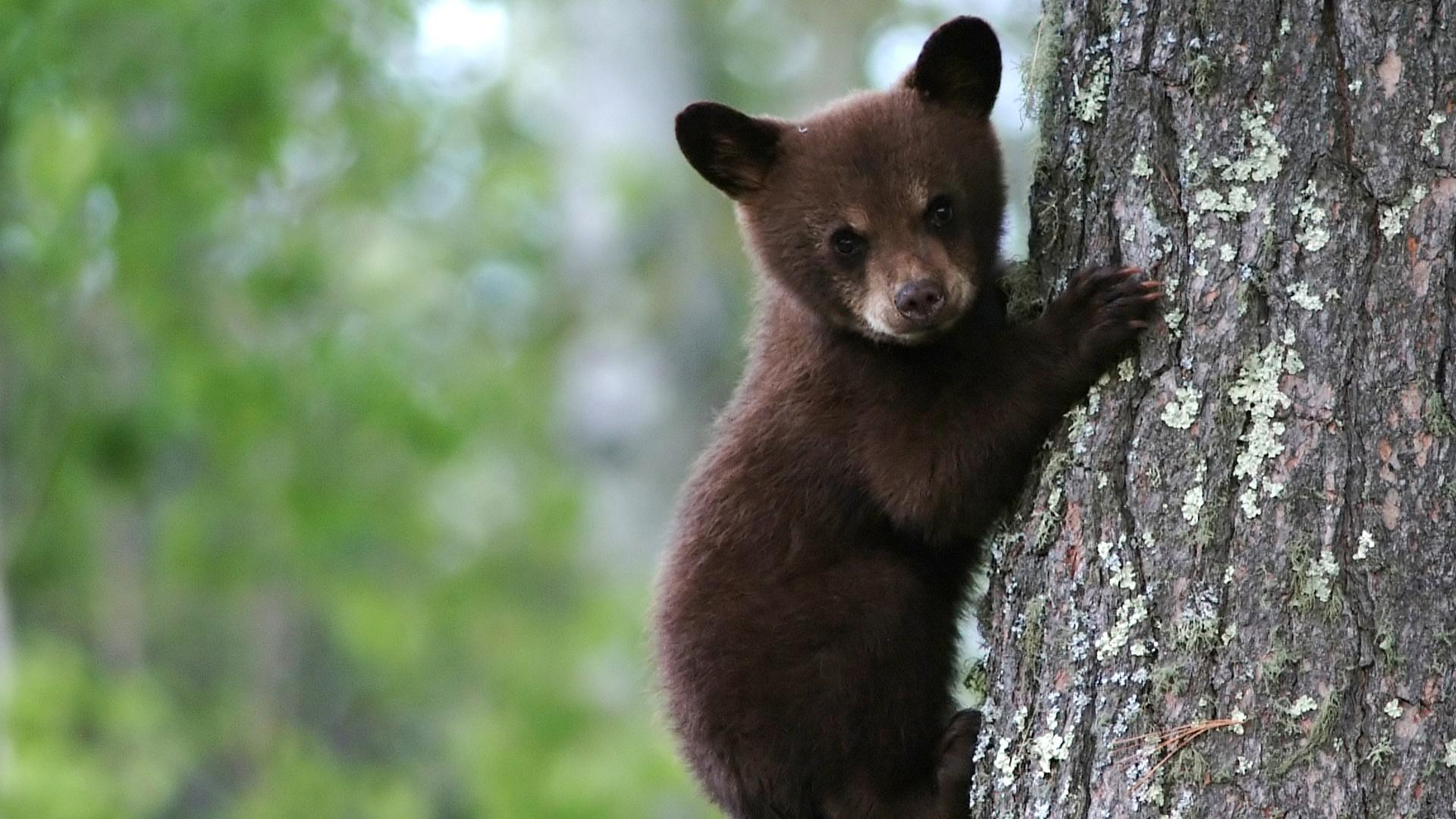In this charming outdoor photograph, a cute little brown bear cub takes center stage as he grips a large tree trunk. The tree, whose thick bark displays reddish and gray tones speckled with green moss, stretches beyond the right edge of the image, illustrating its immense size. The bear cub, climbing vertically with its front paws clasping the tree, gazes directly at the camera with a slightly tilted head, exuding a sense of calm curiosity. His fur is primarily a light medium brown, with darker, almost black ears and a lighter tan shade around his mouth and eyes. The background to the left is blurred, hinting at a lush, green environment with snippets of blue sky peeking through, suggesting a bright, pleasant day in the forest.